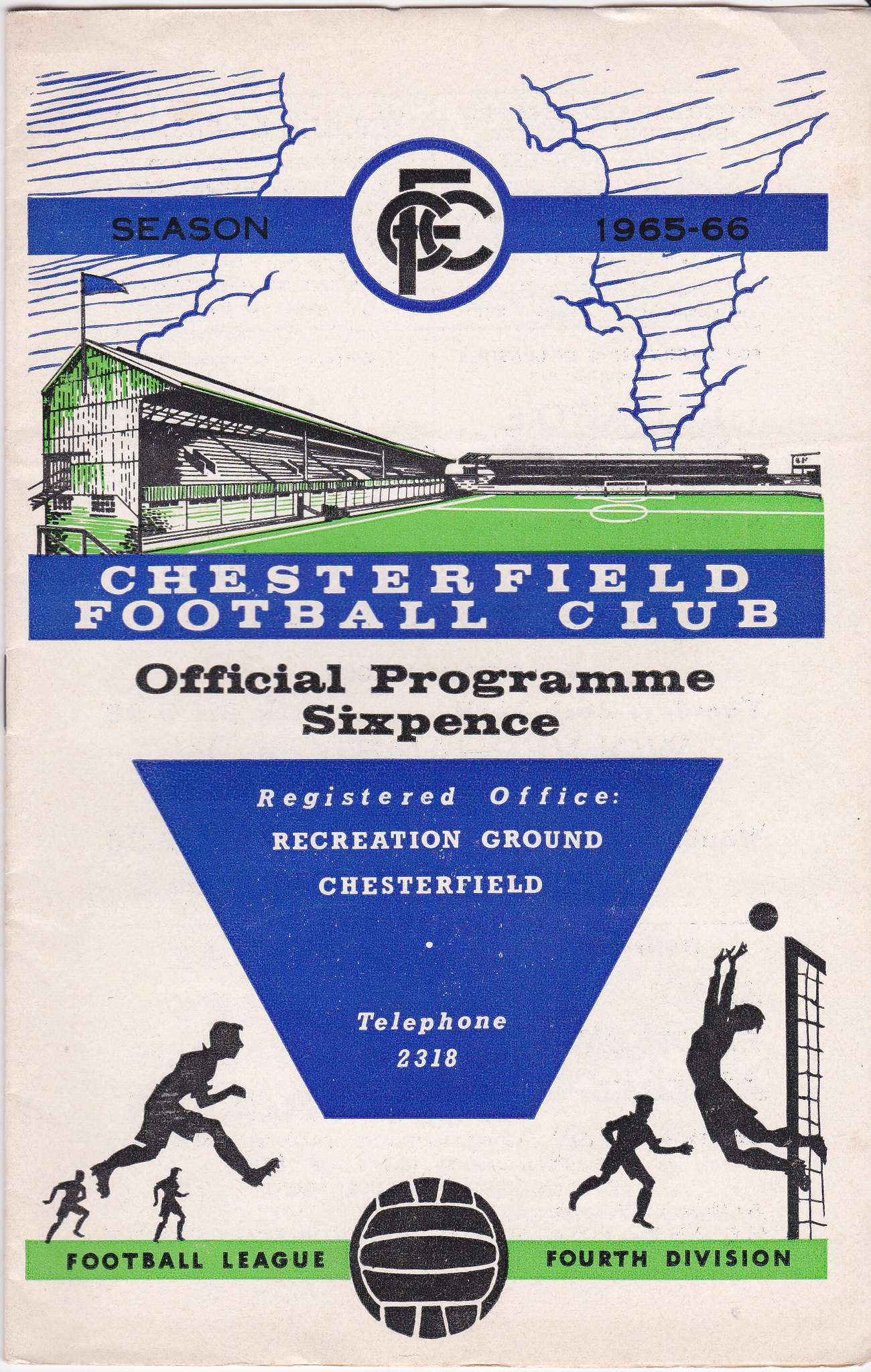The image shows the cover of an official program for the Chesterfield Football Club, dating back to the 1965-1966 season. The background is predominantly white, accentuated by various blue and green elements. At the top, a blue band features black text: "Season 1965-66" with the FCC (presumably Chesterfield Football Club) logo in the center. There are crude outlines, potentially countries, flanking this band on both sides.

Below this, there's a detailed drawing of a soccer stadium with lush green grass, and green and black stands. Beneath this image, another blue band displays "Chesterfield Football Club" in crisp white lettering and labels the document as the "Official Program," priced at six pence.

Sponsorship information follows, indicating the program was produced by the Recreation Ground office in Chesterfield, complete with a telephone number (2318). At the bottom, a thin green strip contains text on both sides—"Football League" on the left and "Fourth Division" on the right—framing a central illustration of a soccer ball. Scattered around the cover are various black-and-white drawings, including silhouettes of soccer players in action and a goalie making a save at the net on the right.